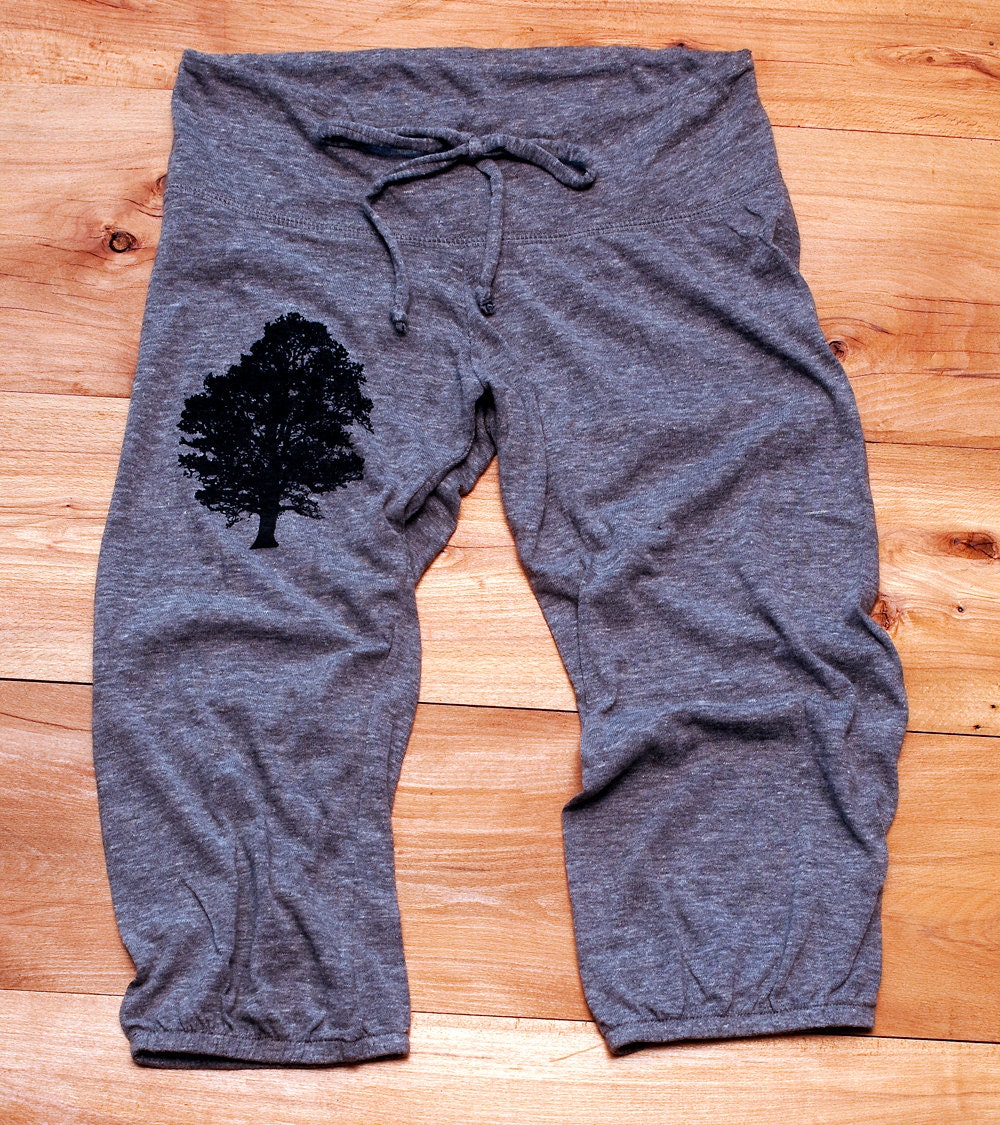The photo captures a close-up of a pair of sweatpants lying on a light, unfinished wooden surface, which could either be a table or a hardwood floor. The wood background features visible knots and a natural, reddish-brown hue. The sweatpants dominate the image, taking up most of the frame and are centered within the shot. These pants are gray and appear slightly crumpled and folded, with a drawstring tied in a neat bow at the waist. They seem to be high-waisted and likely designed for women, suitable for leisure activities or gym wear. A detailed black silhouette of a tree adorns the left thigh, characterized by a short trunk and an abundance of branches and leaves. The pants are made from a stretchable material, especially around the leg openings, emphasizing comfort and flexibility.